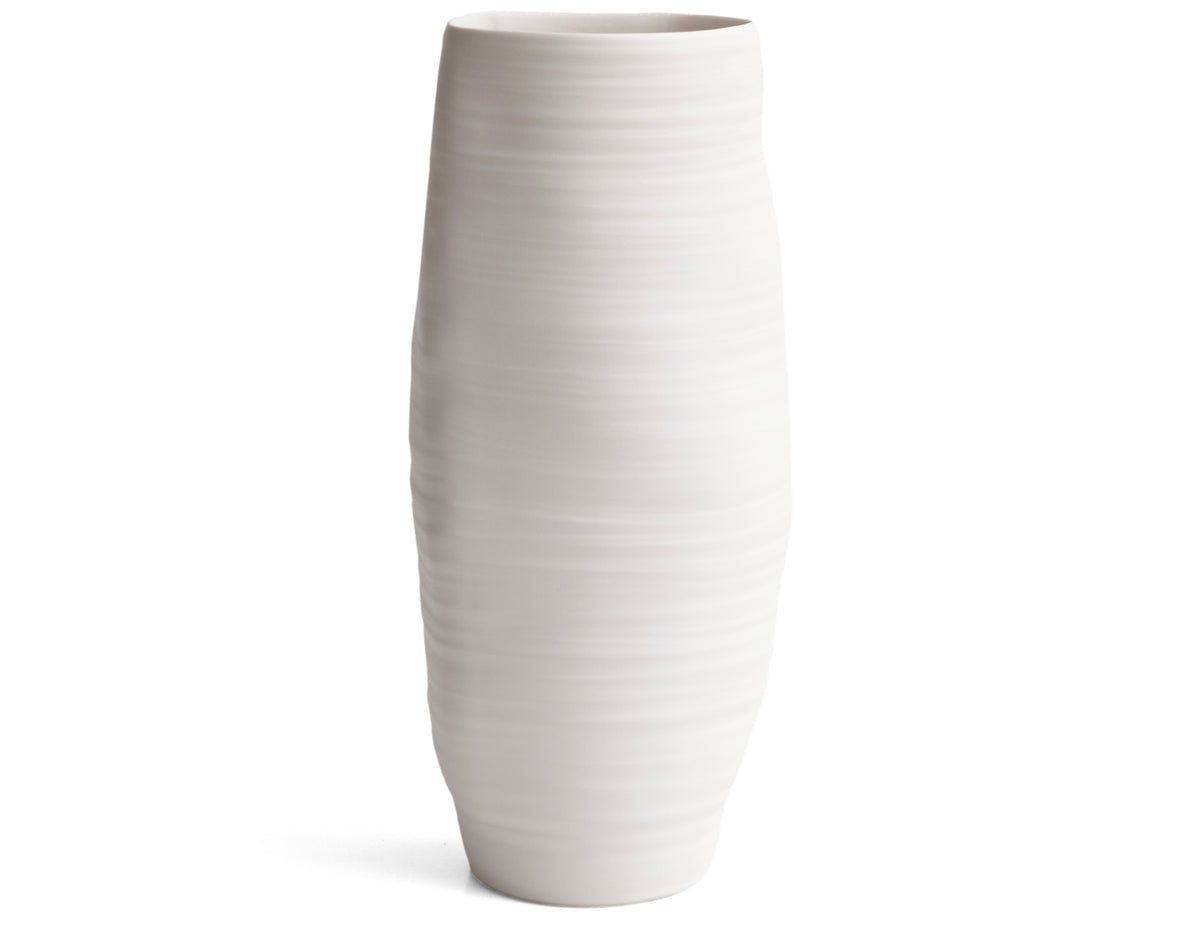The image depicts a tall, narrow cylindrical clay vase set against a plain white background, which almost blends with the vase's light color, giving it a slightly ethereal appearance. The vase, approximately 12 inches tall, is primarily an off-white or pale white with subtle swirled patterns and a very light pink hue that intensifies slightly towards the top, resembling a soft cotton candy shade. The vase features visible lines from the molding process, adding to its handmade look, and a delicate taper from the wider center down to the narrower base and top, both being just under an inch in diameter. It has an uneven, lopsided surface with slight lumpiness, particularly around the midsection, and is encircled by rings formed during its creation. The bottom-left area of the image shows some shadowing, hinting at the vase's three-dimensional form. The vase is empty, making it ideal for long-stemmed plants that would complement its height and cylindrical shape.